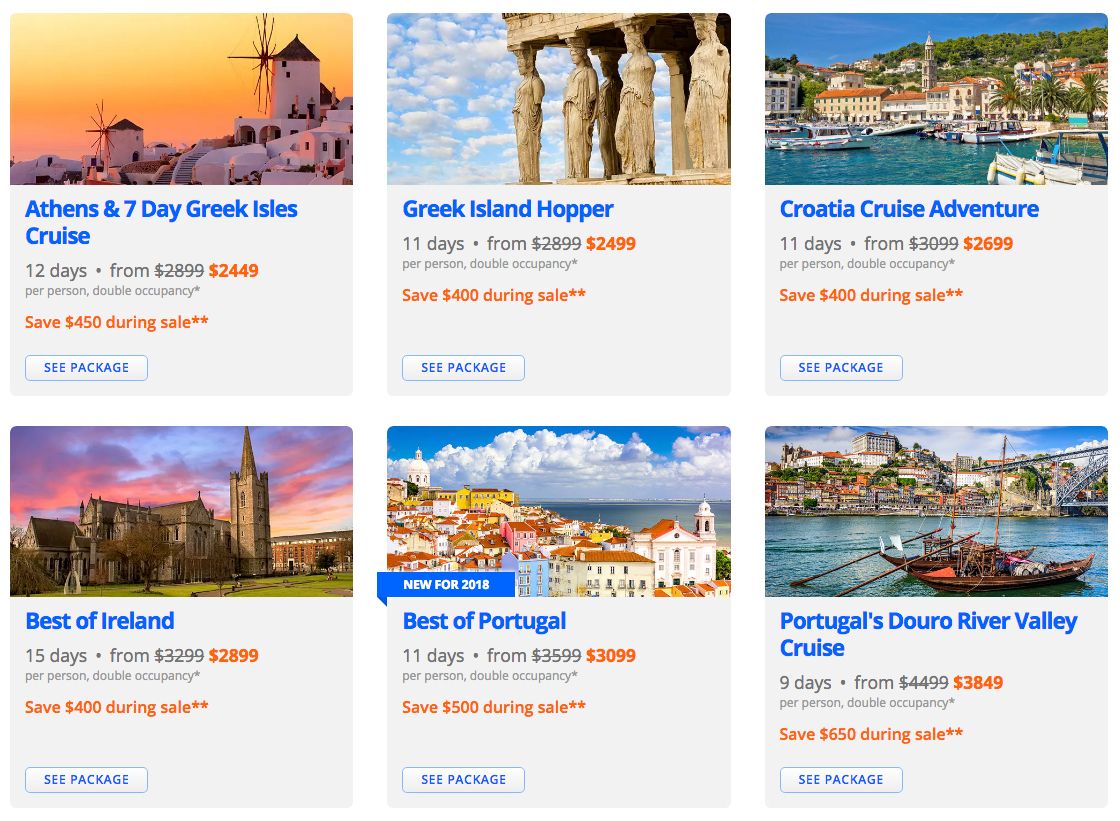The image features a travel advertisement prominently displayed on a web page or app, showcasing six enticing international vacation packages. The origin of the website remains unspecified. Each advertised vacation is depicted with a small, inviting photograph, followed by the vacation title beneath it. Below each title, the duration of the trip and the price are presented, with a clickable button to view further details about the package. The six vacations featured are:

1. **Athens and Seven Day Greek Isles**
2. **Greek Island Hopper**
3. **Croatia Cruise Adventure**
4. **Best of Ireland**
5. **Best of Portugal**
6. **Portugal's Douro River Valley Cruise**

All listed prices have been visibly struck through with a black line, highlighting a special sale price in bold, eye-catching orange, indicating that each of these luxurious vacations is currently available at a discounted rate.